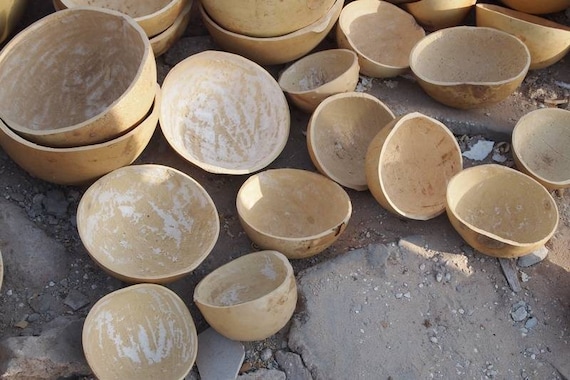In this outdoor scene, the photograph showcases a collection of handmade, light brown bowls, reminiscent of coconut shells or gourd husks, hollowed out and scraped clean. These bowls, some of which have a white powdery residue on their interiors, are scattered and stacked across a messy, rocky, and dirt-laden surface. On the upper left, a couple of bowls are neatly piled in pairs, while others of varying sizes are dispersed throughout the image, resting on what appears to be a rough, gravelly area. The setting suggests a rustic, possibly makeshift work area, adding a raw, organic texture to the scene.